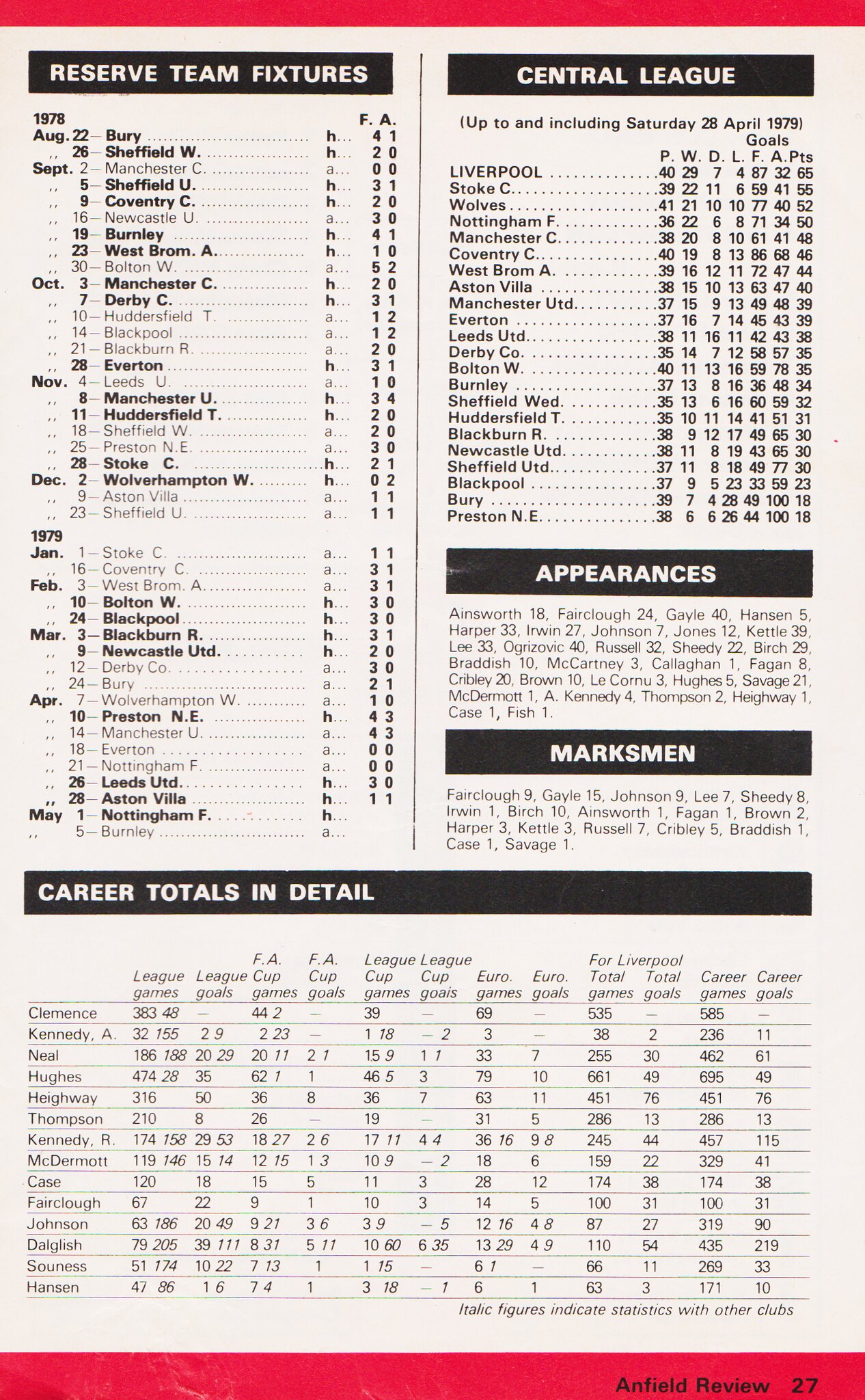The image depicts a detailed page from a magazine, likely the "Anfield Review," with a focus on sports statistics from 1978. The page, numbered 27, features a small red border at the top and a larger red border at the bottom, with illegible text and a number in the bottom-right corner. At the page's top, "Reserve Team Fixtures" is prominently displayed in a black rectangle with white letters, listing dates from August 22nd to May 5th in the left column beneath it. Adjacent to this, the "Central League" label appears in another black rectangle, listing various teams along with their win-loss records and associated statistics. Below this section, the word "Appearances" is also highlighted in a black box, followed by a list of player names. Further down, "Marksman" is similarly presented, with additional player names included underneath. At the bottom of the page, "Career Totals in Detail" is showcased in a black rectangle spanning the width of the sheet, followed by a comprehensive table of statistics detailing various columns of numerical data. The overall presentation suggests thorough documentation of team and player performances.